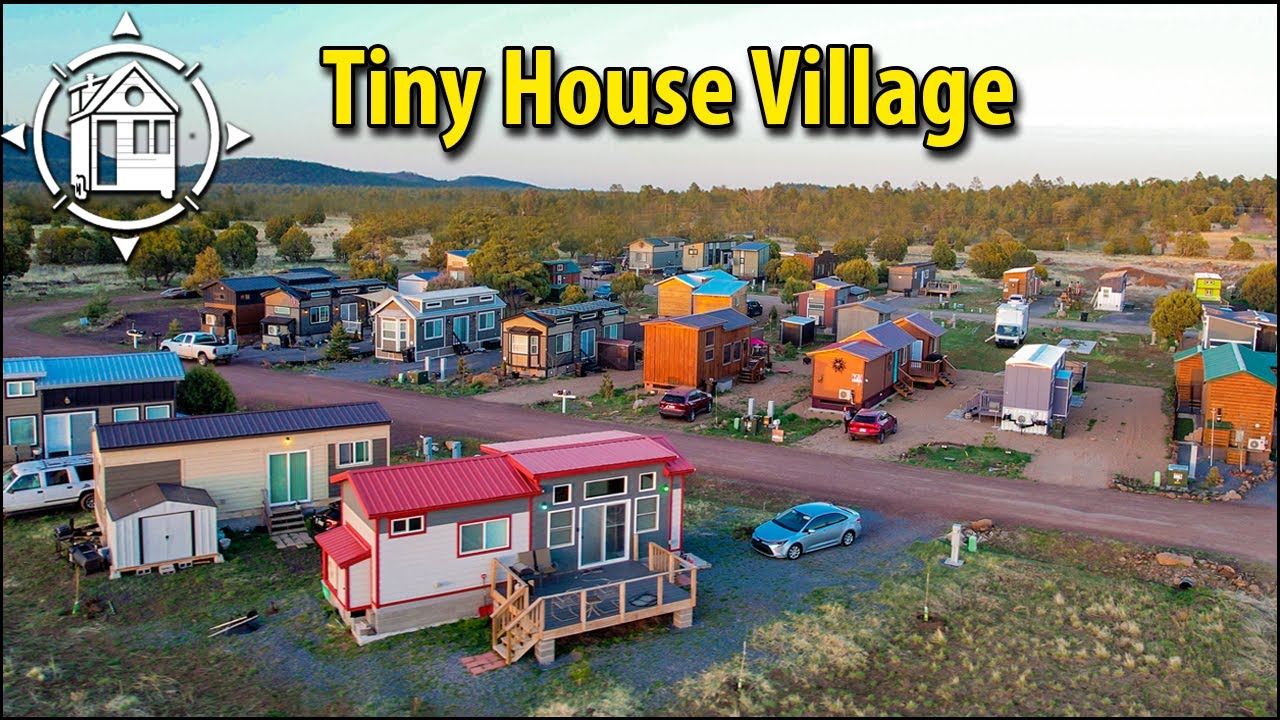The image is a semi-aerial photograph taken from an elevated perspective, approximately three stories high, showcasing a vibrant, tiny house village. At the top of the image, bold yellow text with a black border proclaims "Tiny House Village." In the top left corner, there is a company logo featuring a white circle split into four sections with a small perpendicular line between the curves, resembling rays of the sun, and centered within it, there is an icon of a mobile home. 

The village is neatly organized into three distinct rows of tiny houses, painted in various lively colors such as brown with green, red, or blue roofs, and even one with pink siding and a red roof. These compact homes, resembling motorhomes, are scattered with parked vehicles, suggesting a bustling, lived-in community. In the background, lush greenery and trees interspersed among the houses add to the picturesque setting, making the village appear as a tranquil, innovative residential area. Despite their name, some of the tiny houses seem more spacious than traditional notions, indicating a comfortable living environment within this unique tiny house community.